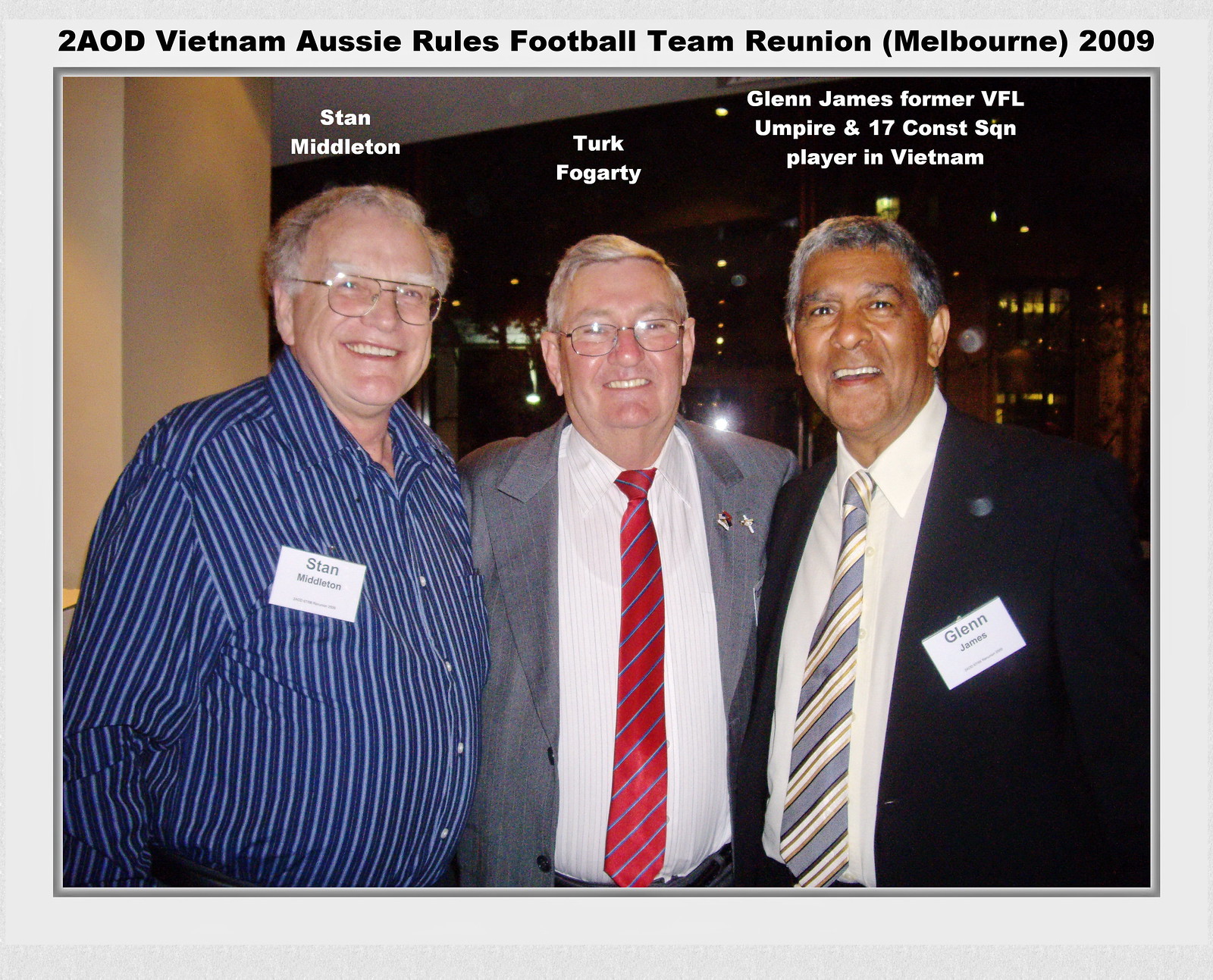The large square image, bordered in gray, captures three men at an event. At the top of the image, in black print, it reads: "2AOD Vietnam Aussie Rules Football Team Reunion (Melbourne, 2009)." Above each man's head, small white text states their names. On the far left, Stan Middleton, slightly heavyset, wears a gray and blue vertically striped button-down shirt and a name tag on his right chest. He has mostly gray hair, wire-rimmed glasses, and is smiling. In the center is Turk Fogarty, dressed in a gray suit jacket paired with a white collared button-down shirt and a red tie adorned with gray diagonal stripes. Turk, with short gray hair and wire-rimmed glasses, also smiles warmly at the camera. The man on the right, Glenn James, has darker skin and salt-and-pepper hair. He dons a black suit jacket over a white collared button-down shirt and a gray tie with white and gold diagonal stripes. A name tag is visible on his left chest pocket. Above his head, the text reads: "Glenn James, former VFL umpire and 17 CONST-SQN player in Vietnam." The event appears to be an indoor reunion, with all men looking directly at the camera and smiling.